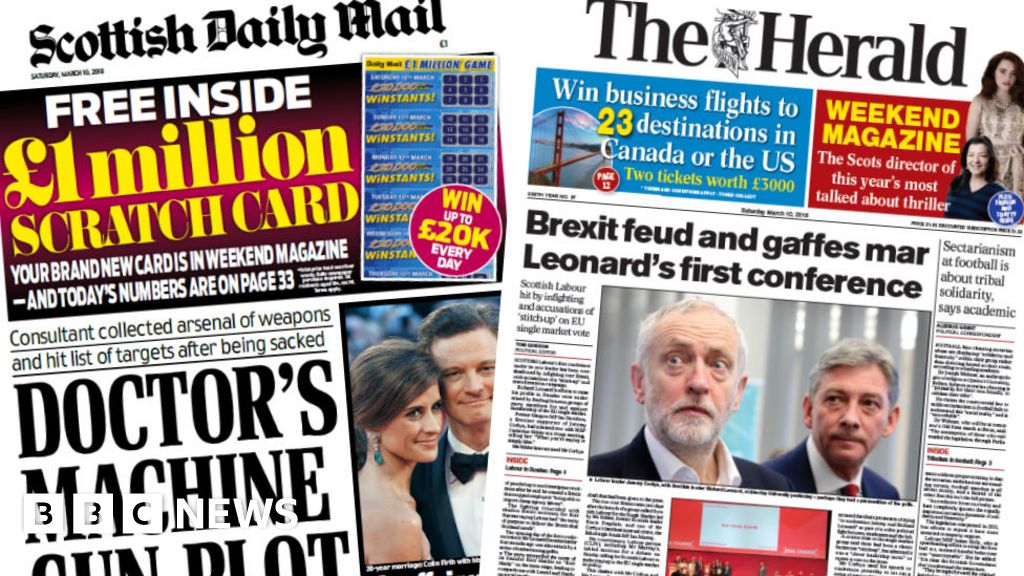In this image, we see the front pages of two newspapers, side by side and equal in size. The newspaper on the left, titled the Scottish Daily Mail, prominently displays its name at the very top center. Below the title is a large rectangular advertisement promoting a "FREE 1 MILLION SCRATCH CARD." This ad also mentions that the brand new card is available in the Weekend Magazine, and today's numbers are located on page 33. Within the ad is a giant scratch card featuring a blue background with yellow writing. Additionally, there is a promotional circle on the bottom left of the ad that highlights "WIN UP TO £20K EVERY DAY," with the words "WIN" and "20K" in yellow. The bottom half of the left newspaper carries a headline that reads "Doctors Machine Gun Plot," and the bottom left corner also includes the logo of "BBC News."

On the right-side newspaper, titled The Herald, the name is clearly visible at the top center. Underneath the masthead is a small rectangular advertisement offering a chance to "WIN BUSINESS FLIGHTS TO 23 DESTINATIONS IN CANADA OR THE U.S." To the right of this ad, there is an entry mentioning the "Weekend Magazine," highlighting the article about the Scots director of this year's most talked-about thriller. In this section, the words "Weekend Magazine" are in yellow text against a red background, drawing attention to the feature.